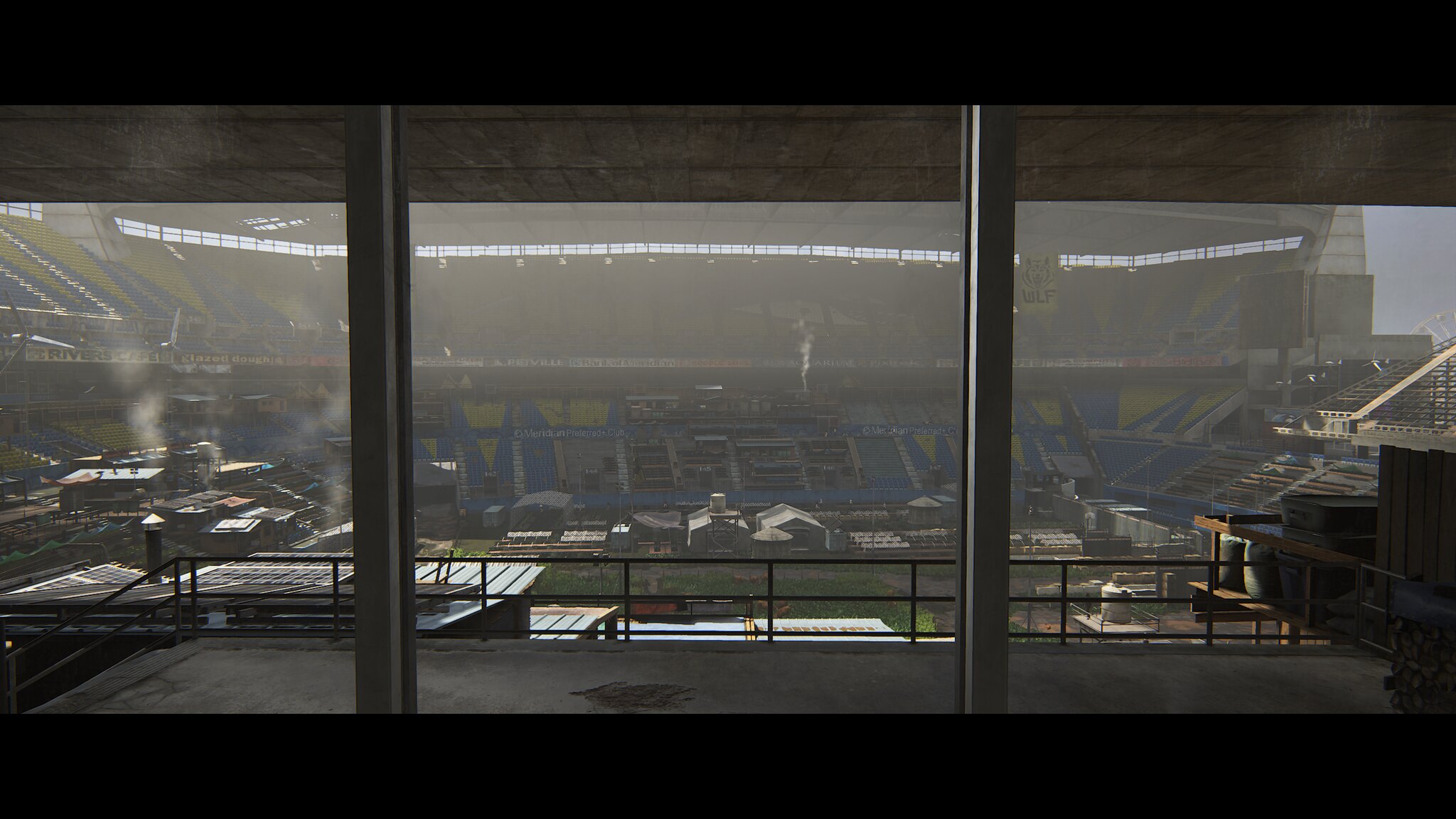**Caption:** 

Captured from within an owner's box, this intriguing image showcases a soccer stadium that has been transformed into what appears to be a shantytown reminiscent of the 1930s Hoovervilles. The once pristine pitch is now dotted with makeshift shacks and small structures, suggesting a post-apocalyptic scenario where people have repurposed the field for shelter. The stadium's multi-tiered stands, adorned with a striking blue and yellow pattern commonly seen in prestigious soccer arenas like those in the English Premier League, have been stripped of numerous seats, further indicating their reuse in the reshaping of this dystopian community. The juxtaposition of the grand stadium architecture against the hastily constructed dwellings creates a compelling narrative of survival and adaptation.